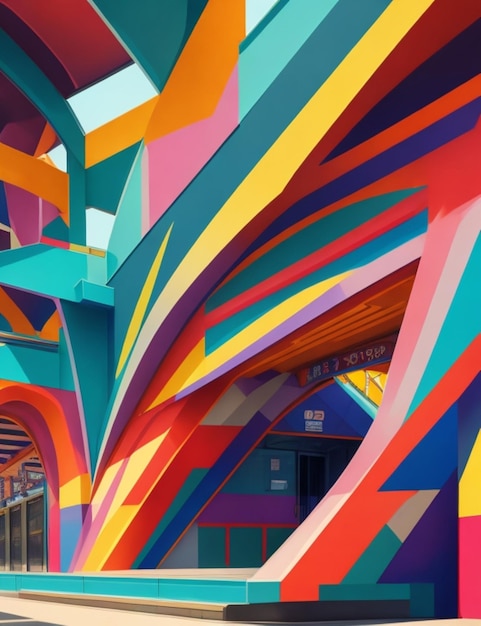The image showcases an art rendering, likely painted or computer animated, of the vibrant and unique entrance to a large building, potentially a train station or a stadium. The entrance, standing about 15-20 feet high, is part of a building that rises approximately 100 feet in height. This colorful architectural marvel features a striking array of bright colors—orange, red, blue, teal, magenta, periwinkle, yellow, light purple, pink, white, and sky blue—arranged in geometric patterns such as rectangles, parallelograms, and jagged edges.

Two prominent archways, with one partially visible, display these vivid colors in distinct sections. The cut-off archway is adorned with magenta and orange hues, transitioning into yellow and periwinkle as it descends. Conversely, the other arch is a collage of light purple, periwinkle, red, orange, pink, white, and sky blue, with variations in shade as it stretches upwards.

This multi-storied structure boasts numerous gaps and areas between its elements, creating a sense of openness and allowing natural light to filter through. The intricate interplay of colors and shapes, along with the angular design elements, lend the building an artistic quality that, while possibly inspired by a real location, exists more as a whimsical creation in this image, devoid of any identifiable text or symbols.